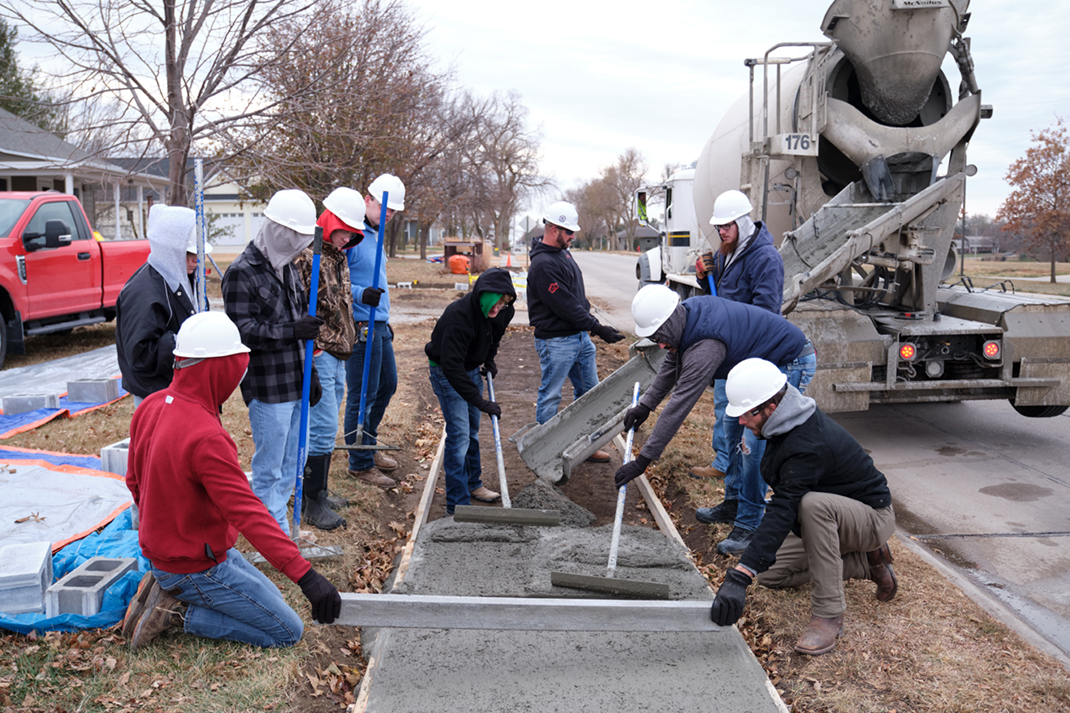In this detailed outdoor photograph, approximately ten workers are depicted constructing a sidewalk adjacent to a completed road where a cement truck actively pours cement. Each worker is equipped with various tools such as brooms and leveling instruments necessary for the cement-laying process. The majority of these workers sport white safety helmets. Notably, one man seen kneeling in the lower left corner, sporting a red hoodie and blue jeans, uses a leveling tool, while another similarly equipped worker, wearing a black hoodie and brown pants, works on the opposite side.

Prominently situated along the left side of the image is a red pickup truck, complemented by a scattering of gray cinder blocks on a blue tarp. Surrounding the area are several trees, many devoid of leaves, and a few houses visible in the backdrop. The ground adjacent to the sidewalk is a mix of yellowish dry grass peppered with brown leaves, though sporadic green patches can be observed.

A notable element in the photograph is the cement truck positioned on the right of the frame, from which gray cement flows through an extended tube into the sidewalk area, delineated by white two-by-fours. The sky overhead is a mix of light blue and white, adding to the overall vividness of the scene.